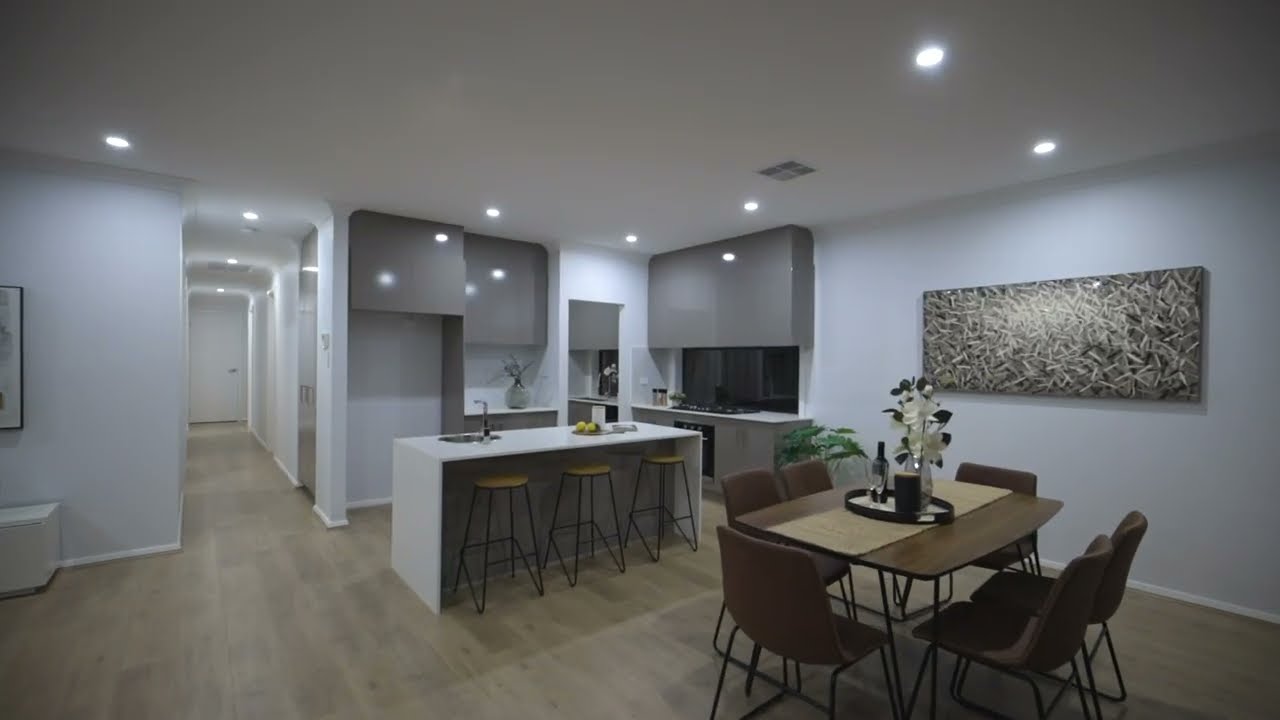This image appears to be a highly detailed rendering of a modern, open-concept apartment interior, exuding simplicity and elegance. The room features smooth white walls highlighted by recessed ceiling lighting that casts a gentle glow. The floor is a light-colored wood, complementing the overall airy ambiance. 

In the foreground, a thin wooden dining table with six leather chairs is prominently positioned to the right. Atop this table, one can find a vase with flowers, a water bottle, and a plate, suggesting a recently set scene. 

The background showcases a sleek, modern kitchen characterized by gray cabinets, white countertops, and a black stove. It appears to be newly constructed or staged, as it lacks a refrigerator. Above the kitchen counter, a window reveals the darkness outside. Noteworthy details include bar stools under a bench seating area, adding both functionality and aesthetic appeal.

The walls are adorned with various pieces of abstract art, including a large rectangular piece and another in a black frame whose details are indistinguishable. Overhead lights enhance the visibility and ambiance of the space, making it feel inviting.

The image also features a hallway leading to a doorway in the background, indicative of the apartment’s spacious layout. The scene blends various colors, including white, brown, green, black, gray, yellow, and tan, creating a harmonious and balanced visual experience.

Overall, the detailed rendering of this modern apartment interior captures an open, well-lit, and tastefully decorated space, seamlessly integrating kitchen and dining areas while highlighting the simplicity and functionality of contemporary design.